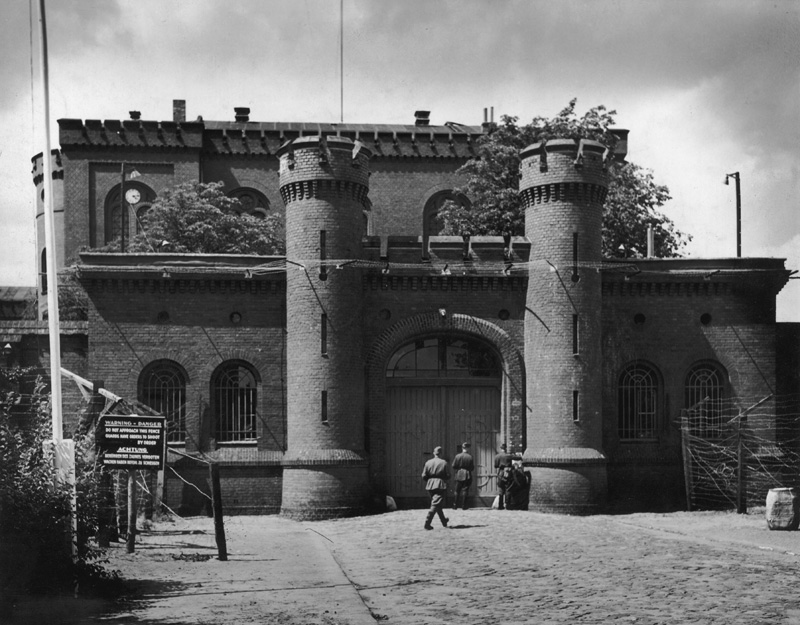The old black and white photograph depicts a brick structure with castle-like features, including two tall pillars framing large wooden doors. The columns have jetted tops, possibly serving as defensive lookouts, enhancing the building's fortress appearance. A barbed wire fence with a "Warning: Danger, Do Not Approach" sign surrounds the structure, suggesting it could be a military compound or prison camp from a bygone era. In the courtyard area, visible behind the entrance, there are two trees and an unflagged flagpole. A cobblestone or brick road, flanked by dirt areas, leads up to the gates, where three men are approaching. The building also has barred windows, consistent with the period and purpose inferred. In the background, partially obscured by the cloudy sky, another large column and some trees can be discerned, contributing to the detailed and somber atmosphere of the scene.